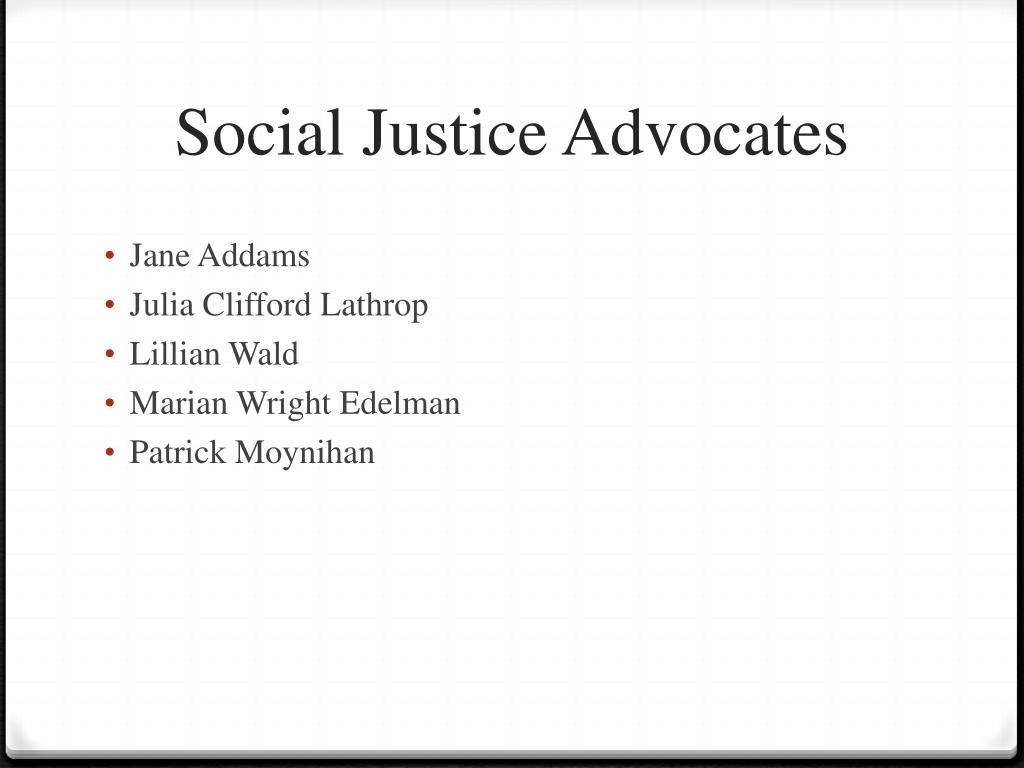The image displays a square panel with black text on a white background, offering a clear and straightforward appearance. At the top center of the panel, the bold black text reads "Social Justice Advocates." Below this title are five names listed in a vertical arrangement, each accompanied by a red bullet point that adds a subtle pop of color against the monochromatic background. The names listed are Jane Addams, Julia Clifford Lathrop, Lillian Wald, Marian Wright Edelman, and Patrick Moynihan. The names are slightly indented towards the left side of the panel. The style of the image resembles a clean, organized list that could be part of an advocacy website or a presentation, with hints of faint lines in the background reminiscent of a notebook page and a black outline framing the panel, except at the top, enhancing its formal appearance.